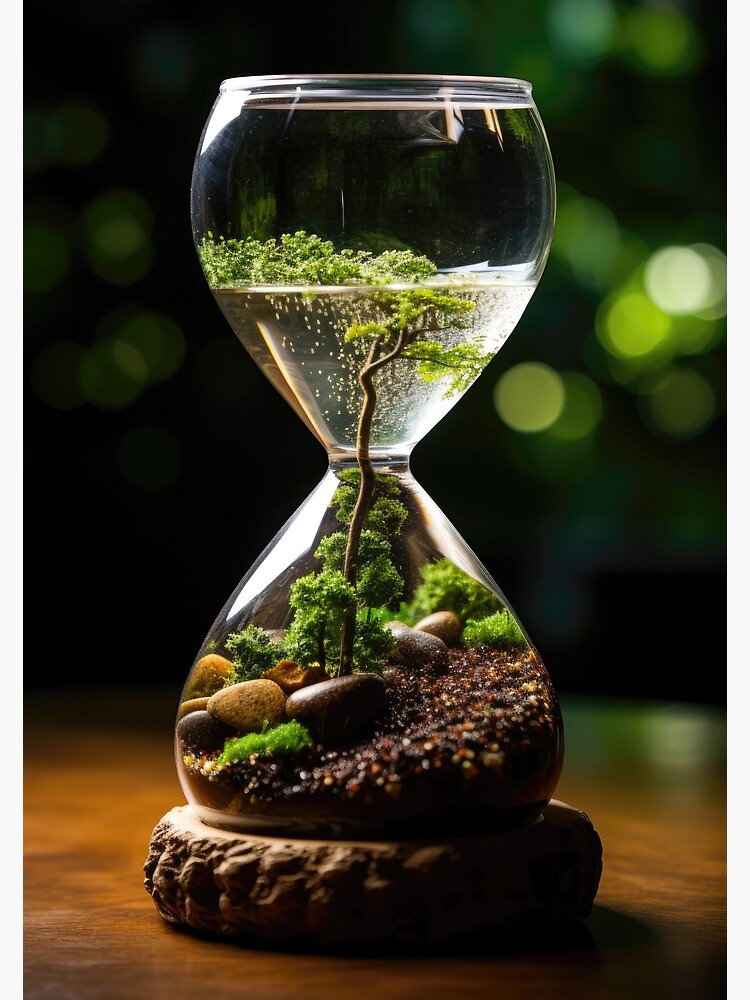The image depicts an artistic hourglass-shaped glass vase, functioning as an aquatic terrarium that evokes a miniature forest scene. The vase, filled about three-fourths with water, is securely nestled on a semi-circular rock or wooden stand placed on a wooden table. Inside the vase, the lower half contains small brown gravel and larger rocks of varying shades of brown, speckled with what appears to be moss. Emerging from this base, a large branch resembling a bonsai tree stretches upwards, piercing through the midpoint of the hourglass and into the upper half, where it is accompanied by clusters of green shrubs and leaves. These branches and foliage create a dense, forest-like environment within the glass structure. The backdrop of the image features a blurred dark green background, accented with light green and whitish circular reflections, directing focus towards the intricate, terrarium-like world contained within the hourglass.